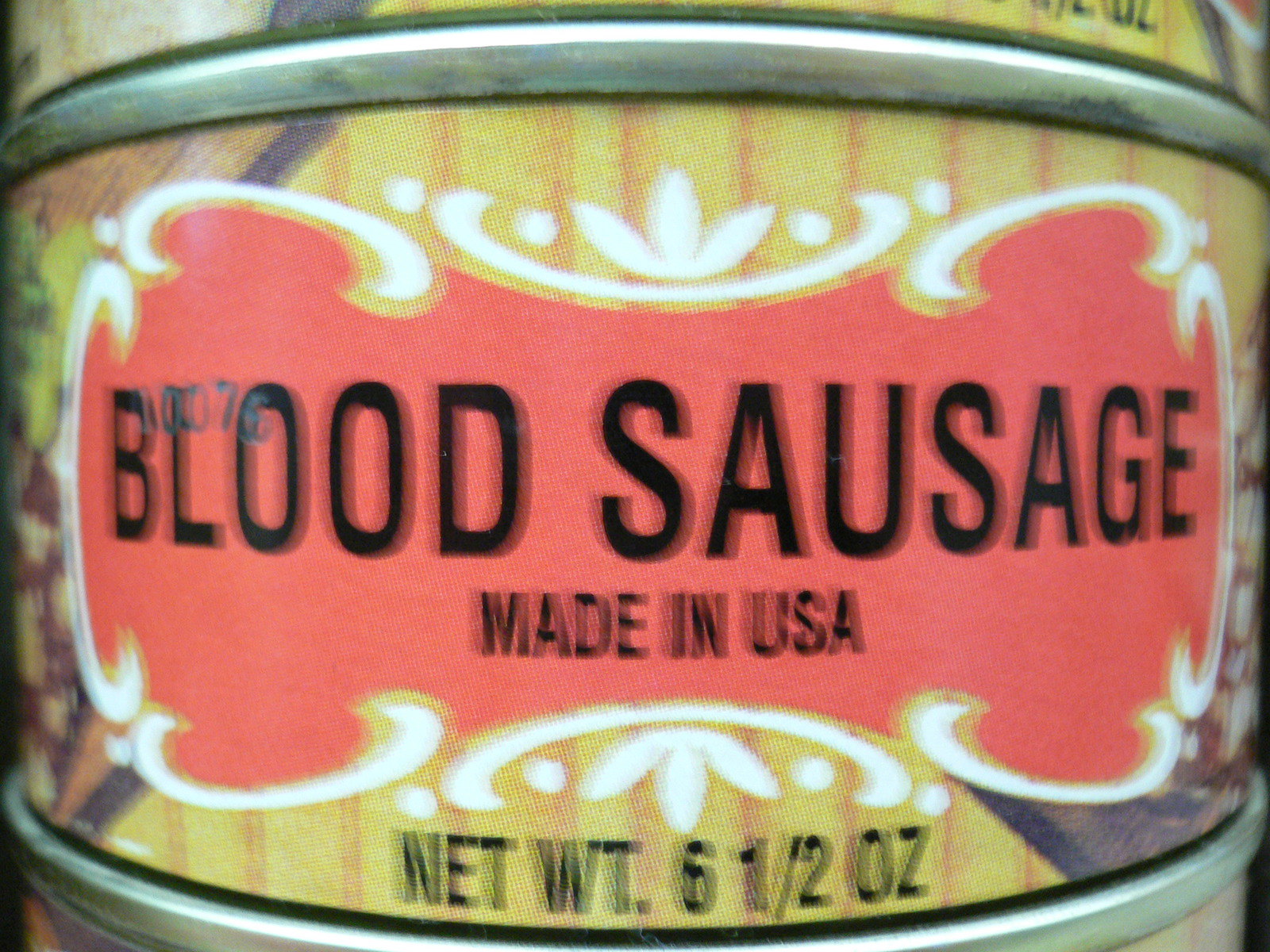This image is a close-up side view of a can of blood sausage stacked among other similar cans. The focus is on the middle can, with the top and bottom cans partially visible. The featured can is small and short, akin to a tuna can, and has a metallic rim at both the top and bottom. The label on the can is primarily yellow with vertical stripes, and it prominently features a red bone-shaped design surrounded by white swirls. In bold black capital letters, the label reads "BLOOD SAUSAGE," with "MADE IN USA" printed underneath in smaller black text. At the bottom of the label, again in black text, it states "NET WT 6 1/2 OZ." The overall arrangement and details suggest the cans are stacked as they might be in a supermarket display. The image is somewhat blurry, but the textual details remain legible.